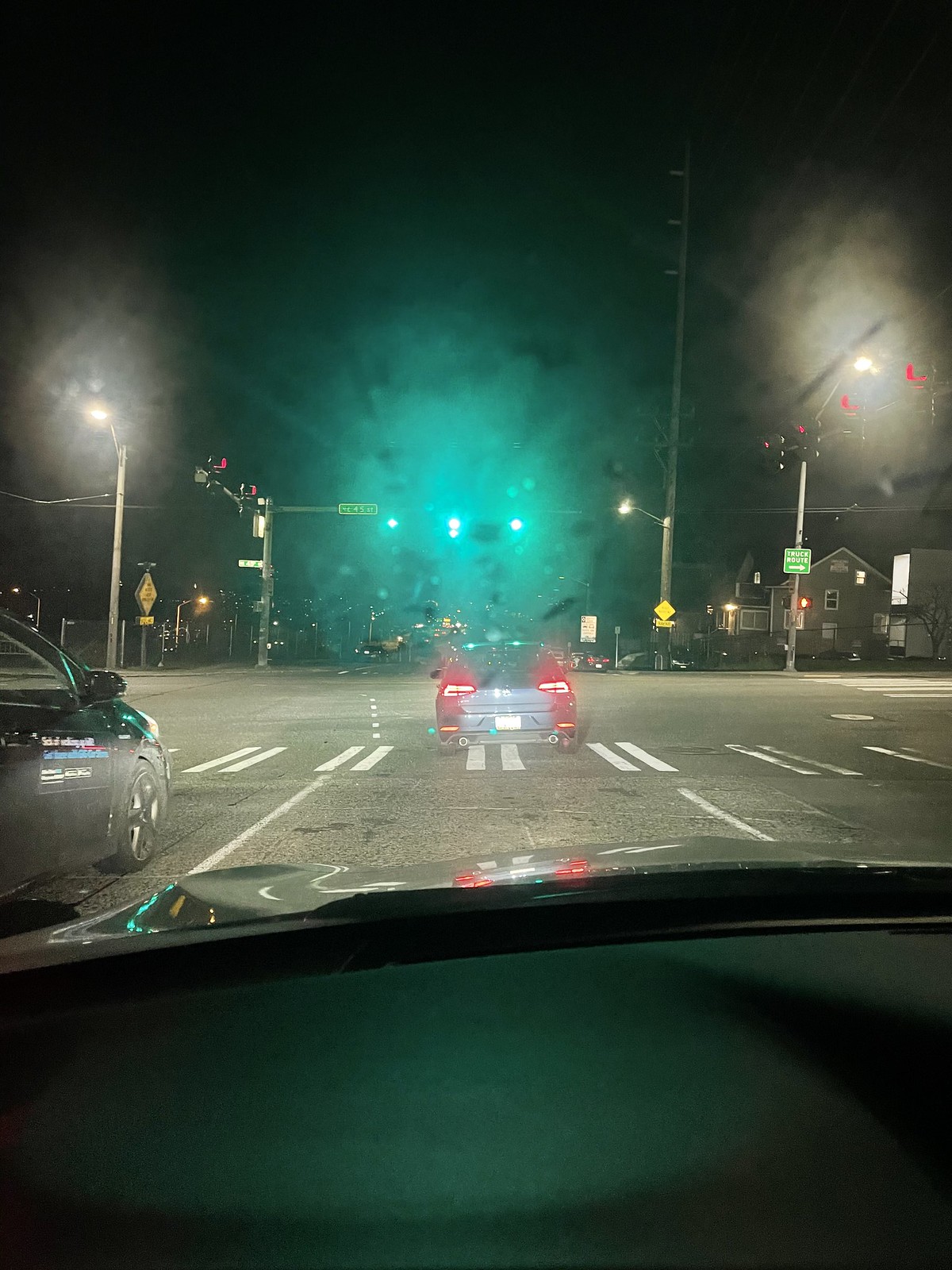The image depicts a night scene captured from a car's dash cam, showing a foggy, four-way intersection. The windshield has a bit of condensation, giving a hazy appearance to the streetlights and creating a soft glow around them. The front edge of the car's hood, which is gray and shiny, is visible along with the dark-colored interior of the dashboard. Directly in front of the car, a dark-colored sedan, possibly blue, has just moved past the crosswalk, with its rear wheels still in the crosswalk. To the left, in the left lane, part of another dark-colored sedan is visible, either with a magnetic sign on its side or reflecting something from a nearby store. The traffic lights in front of the car have turned green, while the lights for the left and right directions remain red. Multiple street signs, including yellow caution and green street signs, are mounted on poles around the intersection. Across the intersection to the right are houses or buildings, illuminated by the bright streetlights and other indistinct lights in the background.